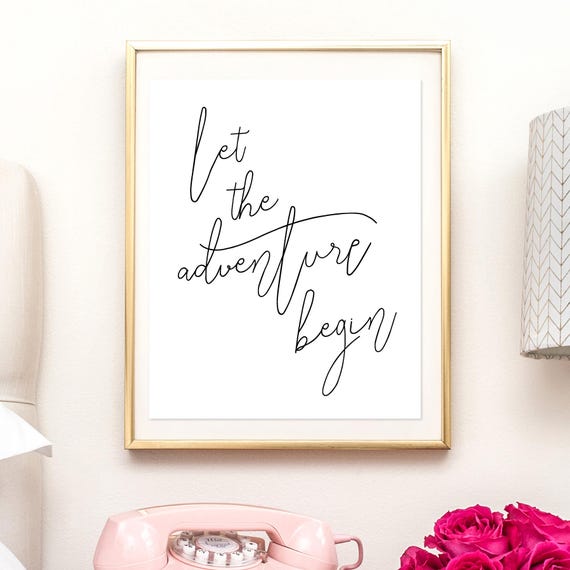The illustration depicts an interior scene featuring a beige-colored wall adorned with a gold-framed picture. The picture, with an off-white background, has black, cursive script that reads, "Let the adventure begin." Below the frame sits a vintage pink rotary phone, positioned on what appears to be a table or shelf. To the bottom right of the frame, there's a bouquet of magenta or pink roses. Also visible in the room is a white lampshade with gold detailing, partially cropped on the right. On the left side of the image, a piece of off-white wooden furniture can be seen, adding to the room's cozy, nostalgic ambiance.